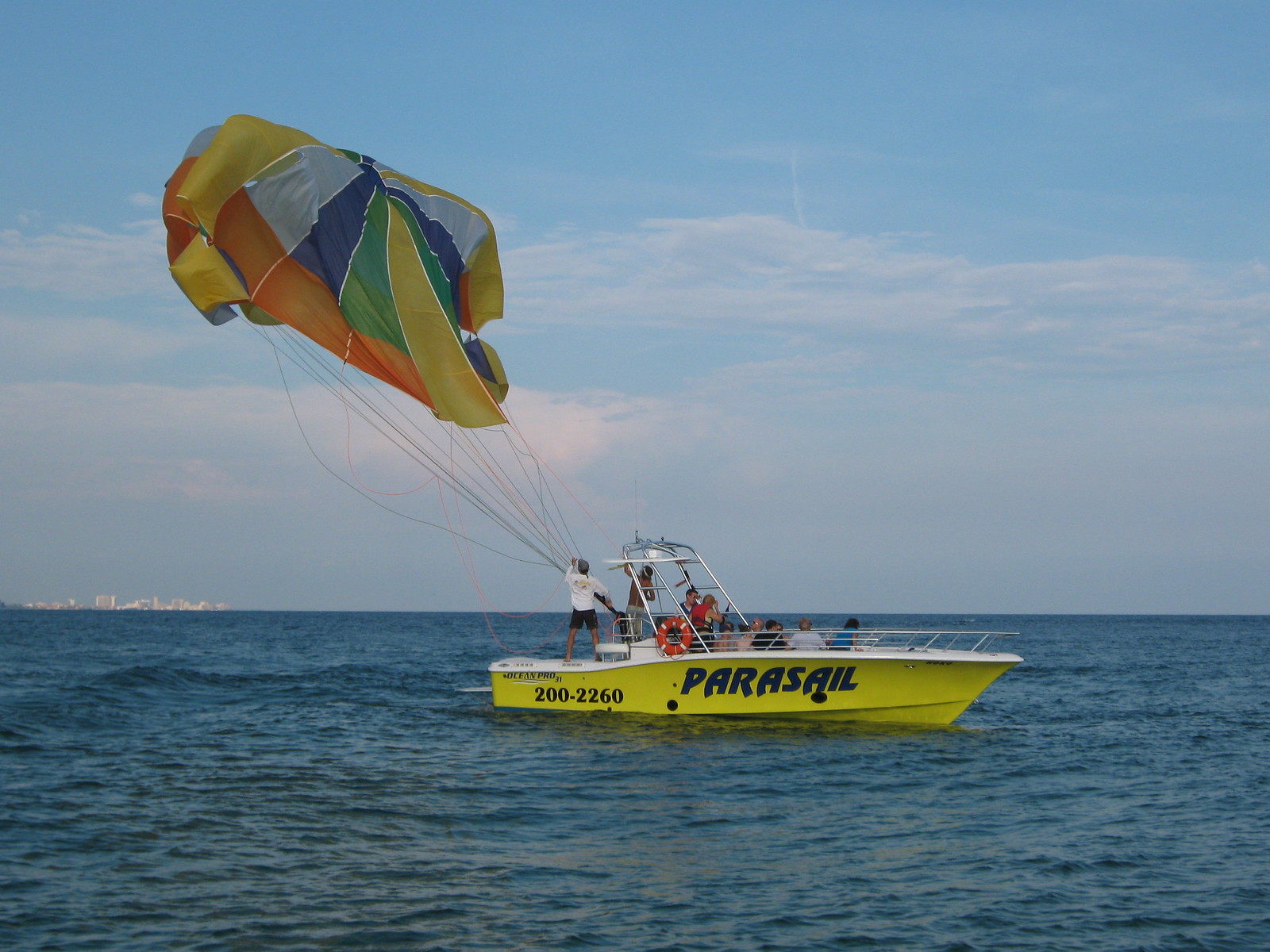This photograph captures an outdoor scene on the ocean under a bright blue sky dotted with faint grayish clouds. In the distance on the left side of the horizon, buildings can be faintly seen. The focal point is a bright yellow boat, labeled "Paracel 200-2260" in black text on its side. The boat features a white trim and is bustling with activity. There are about half a dozen people onboard; most are seated, but a few are standing, including a man in a long-sleeve white t-shirt and black shorts working with a parasail. Another standing person is wearing a red life jacket. The parasail is vibrant, with sections of green, orange, white, blue, and yellow, and floats majestically in the air behind the boat. The dark blue water appears choppy, adding a sense of dynamic movement to this vibrant marine adventure.